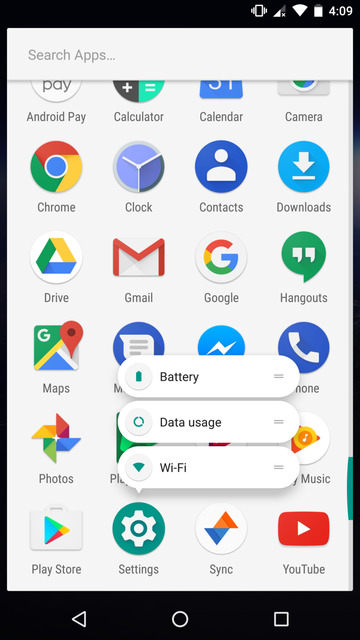The image showcases a cell phone screen with various app icons displayed across six rows. In the top right corner, there are small status icons indicating cellular connection, Wi-Fi signal, and battery life, with a numeric indicator reading '409'. Below these status icons, a search bar labeled "Search apps" is visible.

The first row of icons includes:
1. Android Pay
2. Calculator
3. Calendar
4. Camera

In the second row:
1. Chrome (shown with the Google Chrome logo)
2. Clock (depicted with a clock icon)
3. Contacts (illustrated with an icon of a person inside a circle)
4. Downloads (shown with a blue circle and a downward arrow)

The third row features:
1. Drive
2. Gmail (icon of an envelope with an 'M')
3. Google (a circle with a 'G' in it)
4. Hangouts (a green speech bubble with quotation marks)

The fourth row contains:
1. Maps
2. Two icons with a blue background and an overlaid text box that reads "battery," obscuring the name of these apps
3. Phone

The fifth row presents:
1. Photos
2. Two icons also covered by overlay images
3. Music

Finally, the sixth row displays:
1. Play Store
2. Settings
3. Sync
4. YouTube